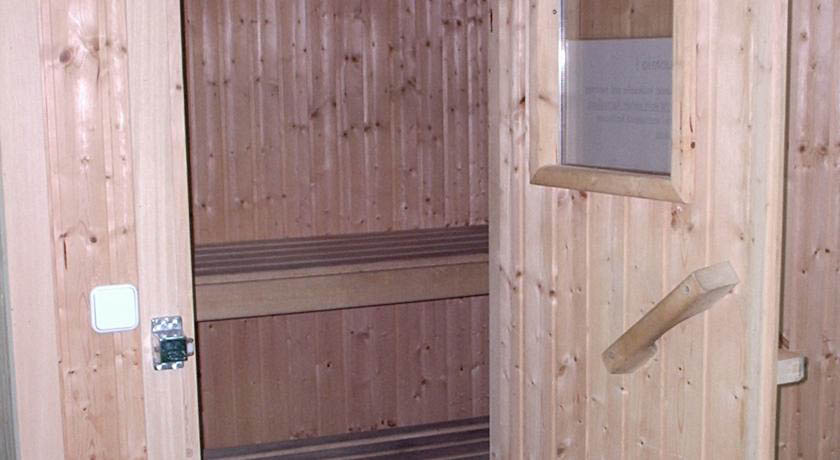The image captures a narrow, wooden room that resembles a small sauna or potentially a pantry. The room is constructed entirely from two types of wood: a darker, reddish-brown wood, possibly like sequoia, and a lighter, oak-like wood. The lighter wood is prominently featured on the door frame and the interior walls, which display vertical wooden slats meticulously fastened together. The entrance to the room consists of a wooden door that is slightly ajar, featuring a window pane covered by a plastic or plastic glass sheet. Inside, there are two wooden benches or shelves, highlighting the functional but minimalistic design typical of a sauna. Noteworthy details include a metallic fastener with a green square on it, which likely serves as the locking mechanism, and a white square on the left side of the picture, which could be a light switch or some form of control panel.